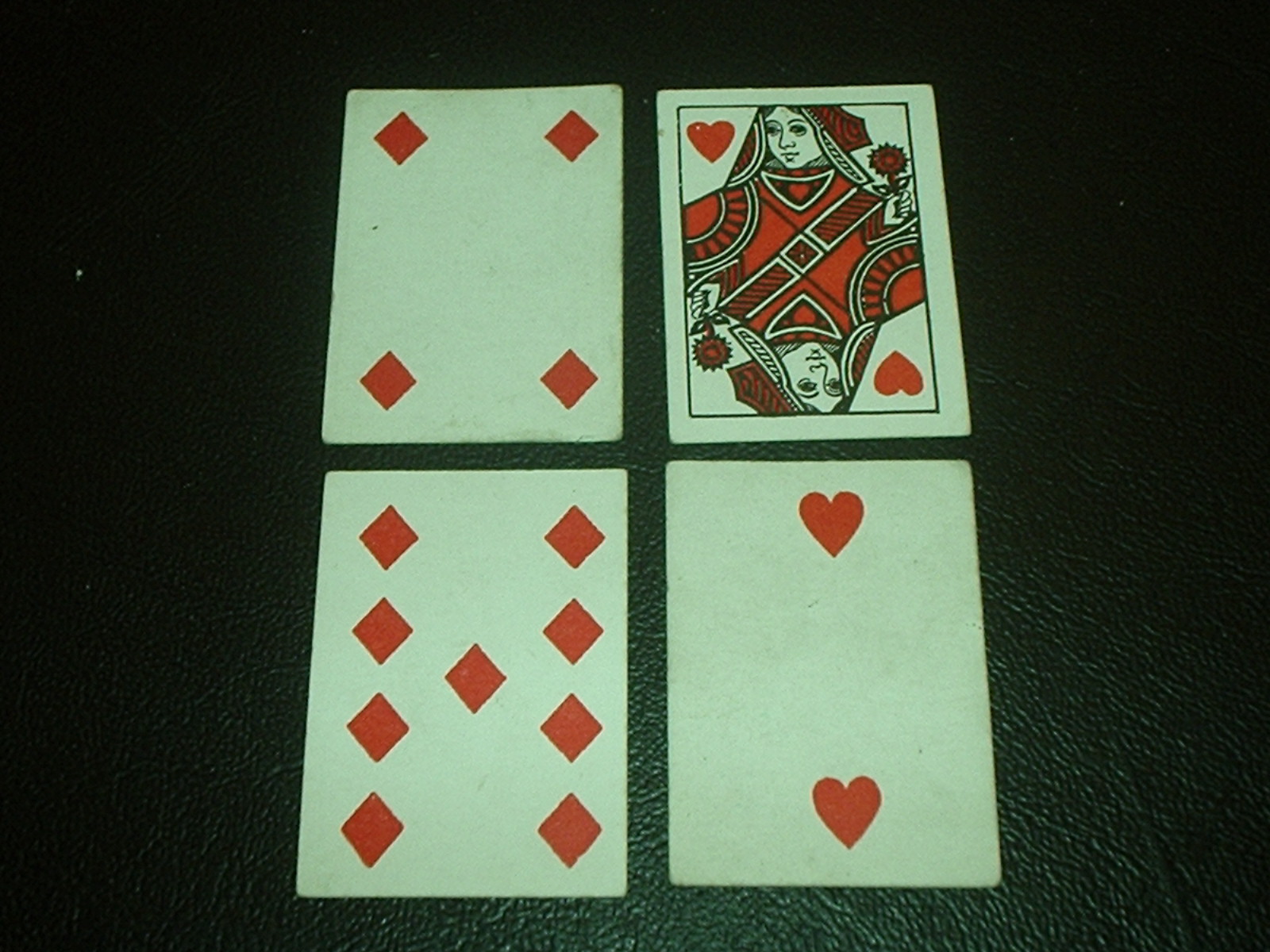The image showcases four playing cards arranged in a grid pattern against a background that appears to be black leather, possibly resembling the material on a couch or chair. The cards are face up and displayed in two rows. The top row consists of:

1. The first card on the top left is a Four of Diamonds, depicted without numerical values, featuring just four red diamond shapes placed in the corners.
2. Next to it, on the top right, is a Queen of Hearts card. This card has the typical Queen portrait, with one Queen image upright and the other upside down, as is traditional in playing cards.

On the bottom row:

1. The bottom left card is a Nine of Diamonds, also without numerical labels. It depicts four red diamonds on each side and one diamond in the center.
2. The bottom right card is a Two of Hearts, similar to the others in that it lacks numeric indicators, displaying a single red heart at the top and another at the bottom.

Each card is displayed on a background that intensifies the stark contrast between the white cards and the luxurious, dark leather texture behind them.